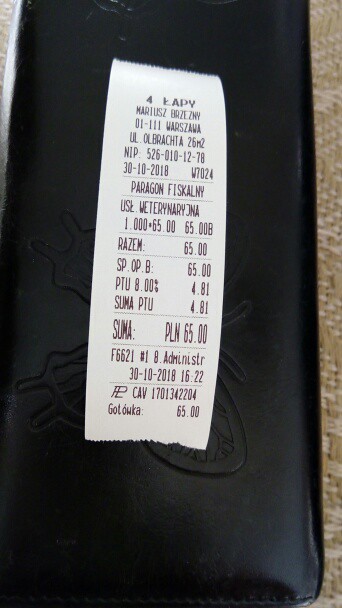The image features a detailed photograph of a white paper receipt with black, computer-generated text, written in a non-English language. The receipt, torn at the top and bottom as if freshly detached from a printer, displays the total amount of 65.00. It rests atop a rectangular, black leather-bound folder, which has stitches along the bottom edge and is embossed with a floral or butterfly design partially obscured by the receipt. This folder lies on a woven, tan, and beige surface, adding texture to the background. The receipt seems to be from a location in Warsaw, Poland, with text mentioning "Paragon Fiskalny" and other localized details such as "KAPY Marius Brezhnev" and "UL Old Brock A26M2." The date on the receipt is 30-10-2018, and additional numbers like F6621 and various codes are visible, giving it an official and detailed appearance.